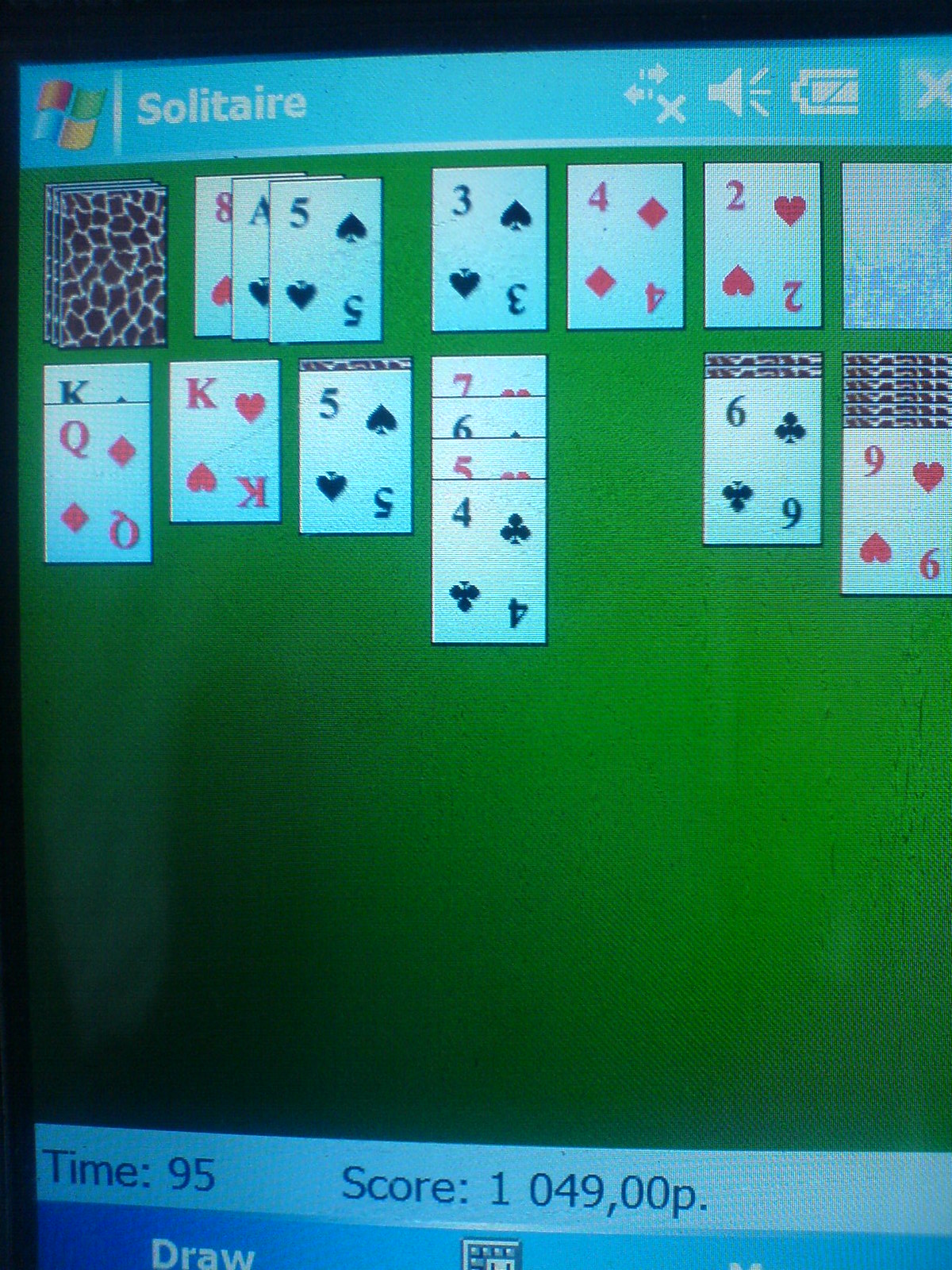The image showcases a computer game of Solitaire on a screen. At the top of the screen, a light blue banner serves as a border, with the word "Solitaire" displayed in white letters. To the left of this banner, there is the iconic Microsoft Windows logo featuring red, green, blue, and yellow colors. To the right, a series of icons are visible, including left and right arrows with an X, indicating potential network connectivity issues, alongside a speaker icon, battery icon, and another X symbol.

The game board itself is green, with cards featuring intricate marbled backs in deep brown and cream hues. The face of the cards displays traditional black and red suits. At the bottom of the screen, another light-colored border contains player information written in black text.